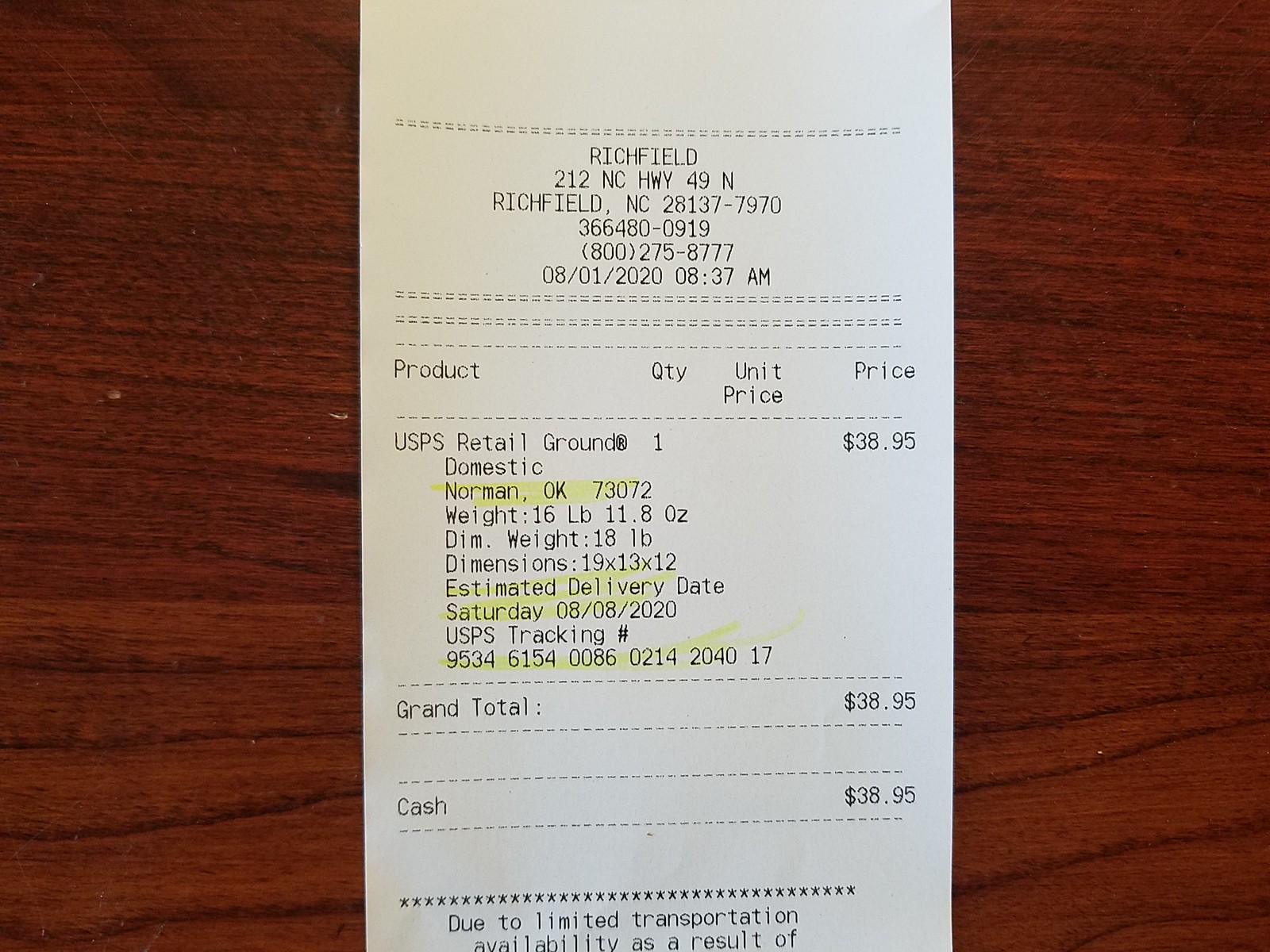This is a detailed photographic image of a long, rectangular white receipt sitting on a dark wooden table with horizontal grain patterns. The receipt appears to be printed with black text, most likely via a thermal printer. At the top, it states "Richfield" along with the address "212 NC Highway 49 North, Richfield, North Carolina, 28137-7970." Below the address, it lists a phone number in brackets "(800) 275-8777." The receipt is dated August 1, 2020, at 8:37 a.m.

This is identified as a shipping receipt from the USPS, as it notes the product as "UPS Retail Ground" intended for a domestic shipment to Norman, Oklahoma. The package weighs 16 pounds and has dimensions of 19 x 13 x 12 inches. The estimated delivery date is August 8, 2020. Following the product details, there's a tracking number: 9534615400860214 204017. The total cost of the shipment was $38.95. 

Notable elements like the recipient, tracking number, and estimated delivery date are highlighted on the receipt. The overall presentation and content provide a clear and comprehensive look at the transaction details.